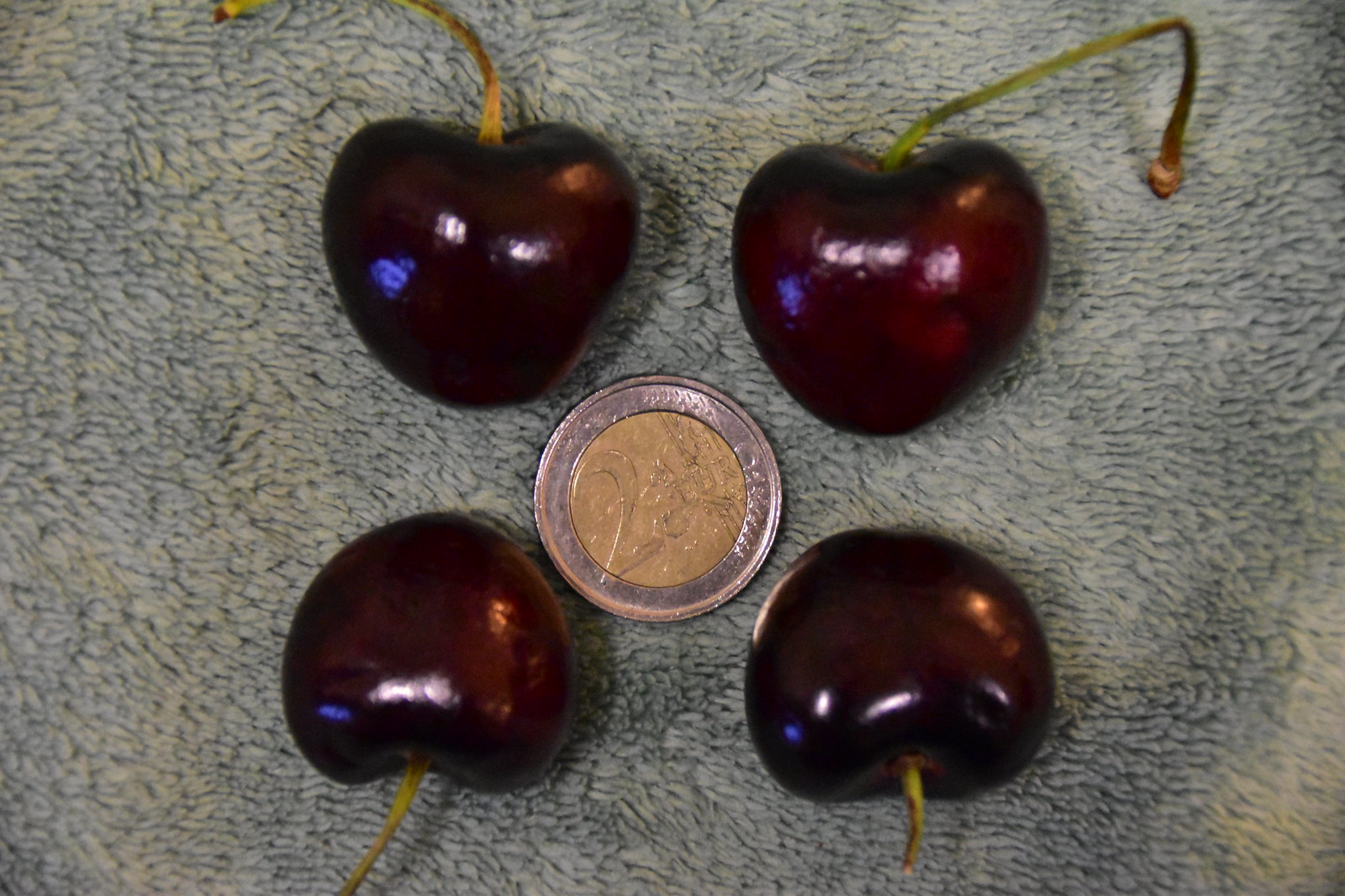An overhead photograph captures a close-up view of four Bing cherries arranged on a soft, light olive-green cloth, possibly terry cloth or a cotton towel. The cherries, which are a deep, dark red, form a square pattern with two cherries on the top and two on the bottom. Each cherry has a stem, varying in color from mostly green to some with gold-tipped ends or browning edges. In the center of the arrangement lies a coin, suggestive of foreign currency, featuring a silver or rose-gold border and a gold center with an unreadable insignia. The overall composition appears to aim for an artistic effect, despite its basic setup.